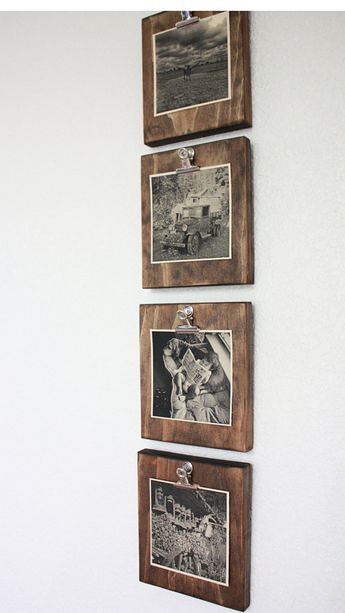The image features a simple, clean white wall adorned with four square, brown wooden panels. Each panel is uniformly brown with vertical streaks of lighter hues and houses a black and white photograph. These panels are vertically aligned in a column and are affixed to the wall by metal hooks with small ties.

The top photograph showcases a vast landscape with dramatic contrasts, displaying clouds over a field, with what appears to be either a silhouette of two people or a four-legged animal in the scene. Below it, the second photograph features an old-time pickup truck, reminiscent of the 1950s, with trees in the background—evoking a vintage, pastoral setting.

The third image captures a tender moment: a toddler leaning against a large, furry dog, holding what looks like a book or newspaper, both seated on a soft surface. The final photograph depicts a large crowd with buildings and a tree in the background. The details are less distinct, suggesting a bustling scene, possibly in a public space or a farm with animals, though the specifics are hard to discern. Each photo's black-and-white aesthetic, combined with the white trimming around them, enhances their classic and timeless appeal.